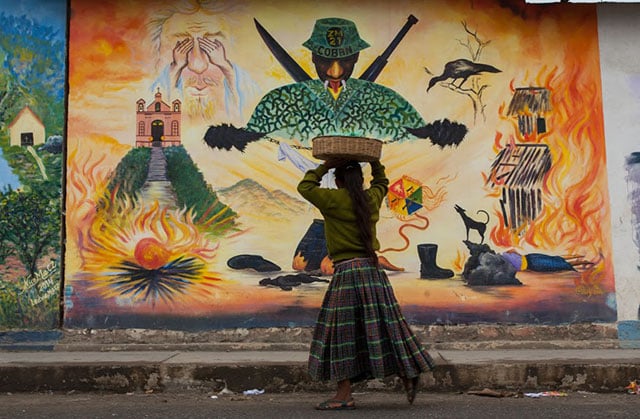This vibrant photograph captures a South American woman with long braided hair, dressed in a green top and a long, dark blue skirt with green horizontal stripes, walking along a sidewalk. She carries a large flat basket on her head, holding it with both hands, and she wears flip flops on her feet. She walks past a detailed and expansive mural covering the entire side of a building. The mural, filled with intense and vivid colors, depicts various scenes of war and its aftermath.

On the right side of the mural, a dog howls next to an owner lying on the ground, surrounded by flames engulfing several huts and houses. In the middle, a man bearing a sword and a gun stands prominently with the letters C-O-B-R-N inscribed on his round hat. To the left, an image of a deity-like figure, possibly God, is shown hovering in the sky, covering their eyes in sorrow above a church with a tree or shrub-lined avenue leading up to it. Below this, there is an ambiguous depiction that might represent a heart on fire. The mural overall vividly conveys the horrors of war through its chaotic and expressive imagery.